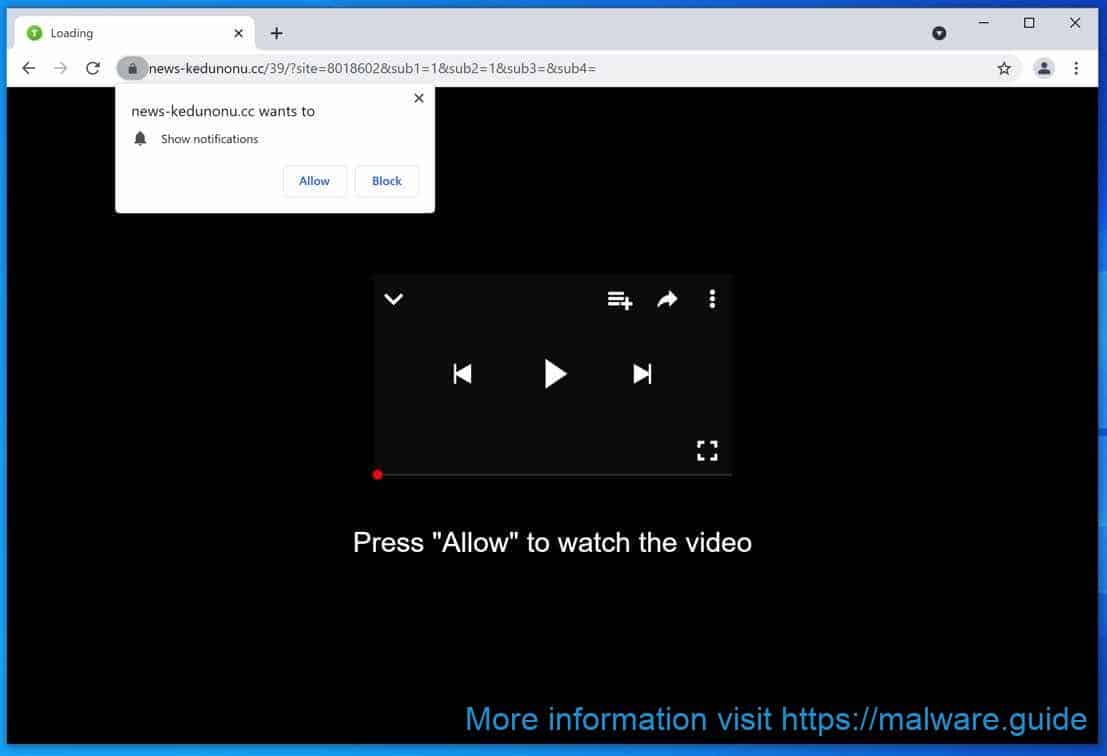The image shows a web browser with a single tab open, displaying a URL that reads "news-kedunonu.cc/39/?site=." The page appears to be loading. A pop-up notification request from the same URL, "news-kedunonu.cc," is present just below the address bar. This notification requests permission to "show notifications" and offers two buttons: "Allow" and "Block," with "Block" in a blue, white-bordered button. There is an 'X' in the upper right corner of the pop-up for closing it.

On the main browser screen, a video placeholder with a black screen is prominently displayed. Below the video, a message prompts the user to "press allow to watch the video." The video controls are visible but inactive, indicating the video has not started playing. The control bar features "backward," "play," and "forward" buttons, with the current position indicator— a red dot— set at the start of the timeline. There is a menu bar represented by three stacked horizontal lines in the top left corner. Additionally, there is a share button with a cross icon at the bottom right of the video section. Each corner of the video control section displays a small white "B."